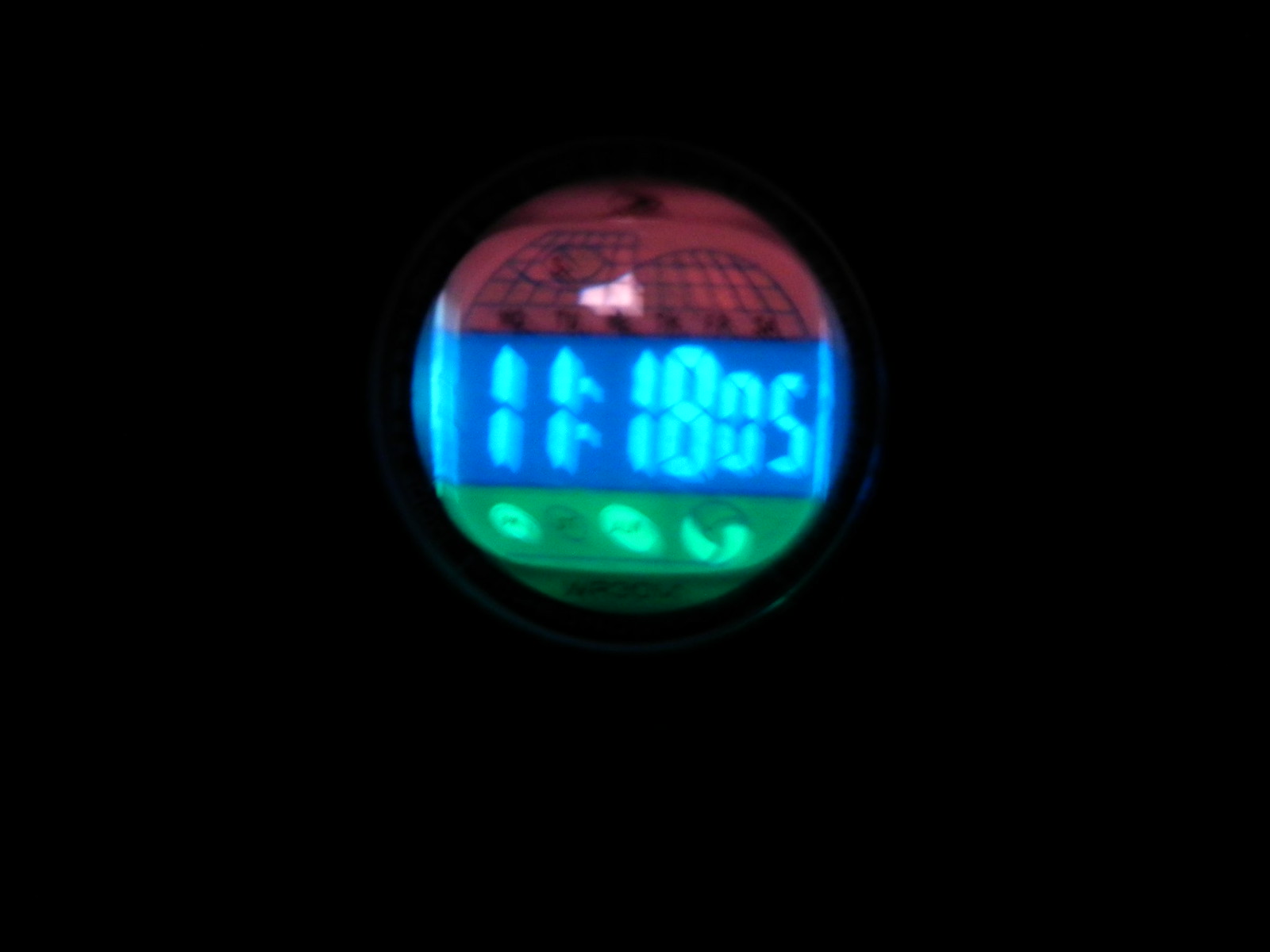The image features the illuminated face of a digital wristwatch, set against a completely black background. The face itself is a slightly squared-off circle, where the top, bottom, left, and right edges are flattened. It is divided into three predominant horizontal sections: a central blue stripe, a wider red stripe at the top, and a narrower green stripe at the bottom. The time 11:18:05 is displayed prominently in traditional LED segments along the blue stripe at the center. Above this, the red section appears to contain a blurry, hard-to-discern logo, perhaps resembling a sketch of the world. Below the blue strip, on the green background, there are several icons: three ovals angled toward the 10 o'clock position, where the left and right ovals are illuminated in green, and a segmented circle on the right with two out of three segments lit up. The entire design is encapsulated within a fine white outer edge, making the face of the wristwatch distinctly stand out against the otherwise pitch-black background.